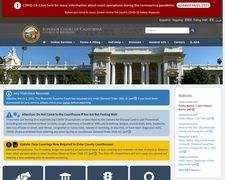The image displays a blurry webpage that is difficult to read due to the small and unclear text. At the top of the page, there is a bright red banner with white text. Below it, a dark gray banner spans across the page with more white text on the right side. Further down, a thicker, lighter gray banner features what appears to be an official seal, suggesting a government affiliation. Adjacent to the seal, white text is present, and a white search bar is located on the far right of this banner.

Continuing down the page, there is a navy blue ribbon that extends horizontally, filled with white text. Below this ribbon, the main visual element is a photograph of an ornate stone building. This building, characterized by its multiple columns and numerous windows, likely represents an important government structure or a museum. The building is bathed in sunlight, set against a bright blue sky.

The lower part of the webpage is divided into various horizontal boxes of different colors, each containing different pieces of information. These boxes are organized in a sequence: a bright blue box at the top, followed by a light gray box, and finally, a bright yellow box at the bottom.